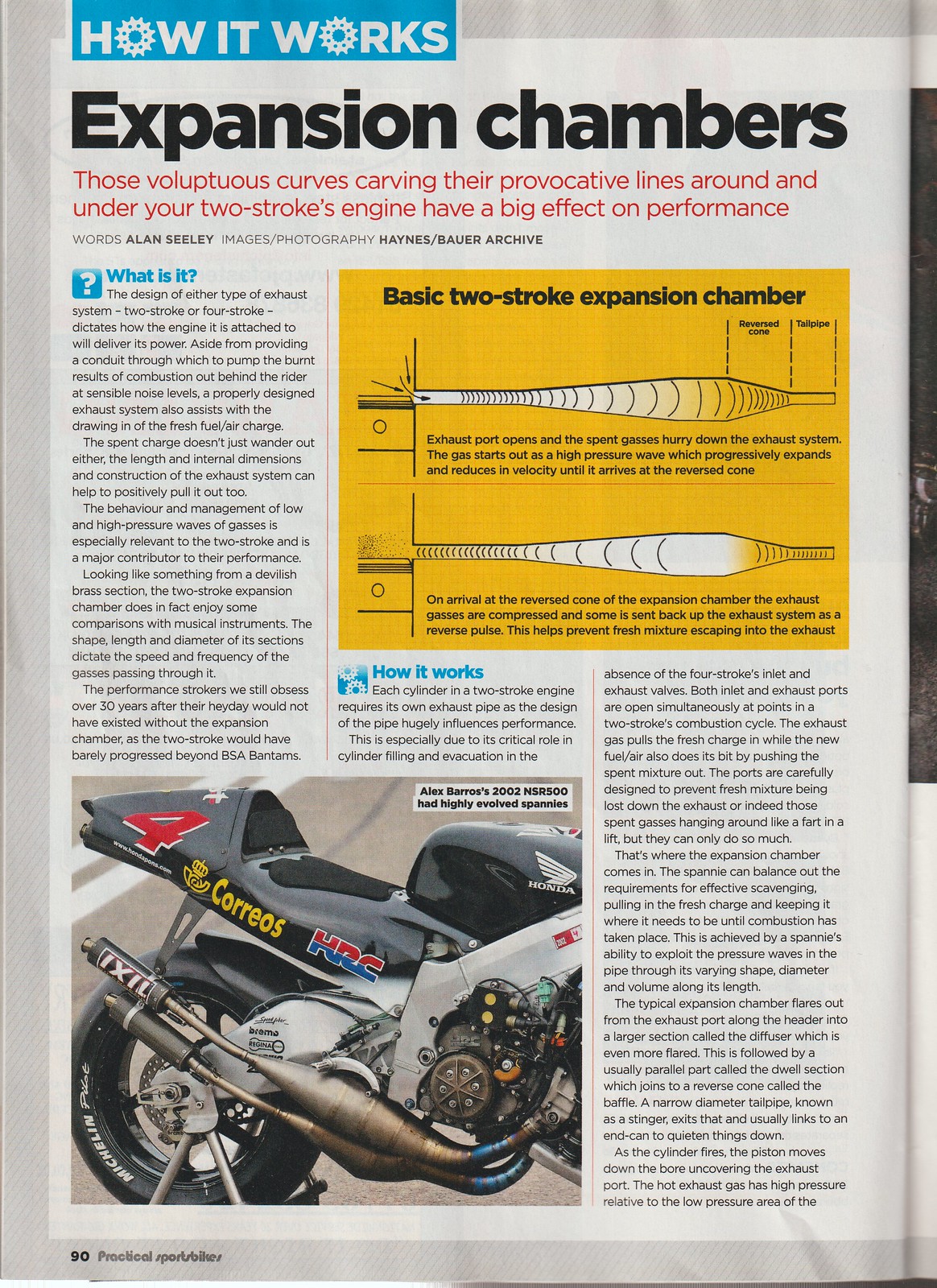This image is a photograph of a magazine page explaining how an internal combustion engine works, particularly focusing on expansion chambers. The page is predominantly black and white with sparse color highlights. At the top left, a blue rectangle features the title "How It Works," with the letters 'O' in "How" and "Works" creatively depicted as gears. The main heading at the top of the page reads "Expansion Chambers" in black letters. Below this heading, in red text, there's an intriguing description: "These voluptuous curves carving their provocative lines around and under your two-strokes engine have a big effect on performance." Towards the upper right side of the page, there is a yellow rectangle containing a graphic that is labeled "Basic Two-Stroke Expansion Chamber," illustrating how the component functions. The bottom left corner of the page showcases the rear end of a black and silver racing motorcycle. The article, written by Alan Seeley and accompanied by images and photography from the Haynes and Bauer Archive, spans across page 90 of the magazine. A caption within the article notes that Alex Barro's 2002 NSR 500 motorcycle features highly evolved expansion chambers, referred to colloquially as "spannies." The rest of the page is filled with detailed text and additional images discussing the technical aspects and performance implications of expansion chambers.